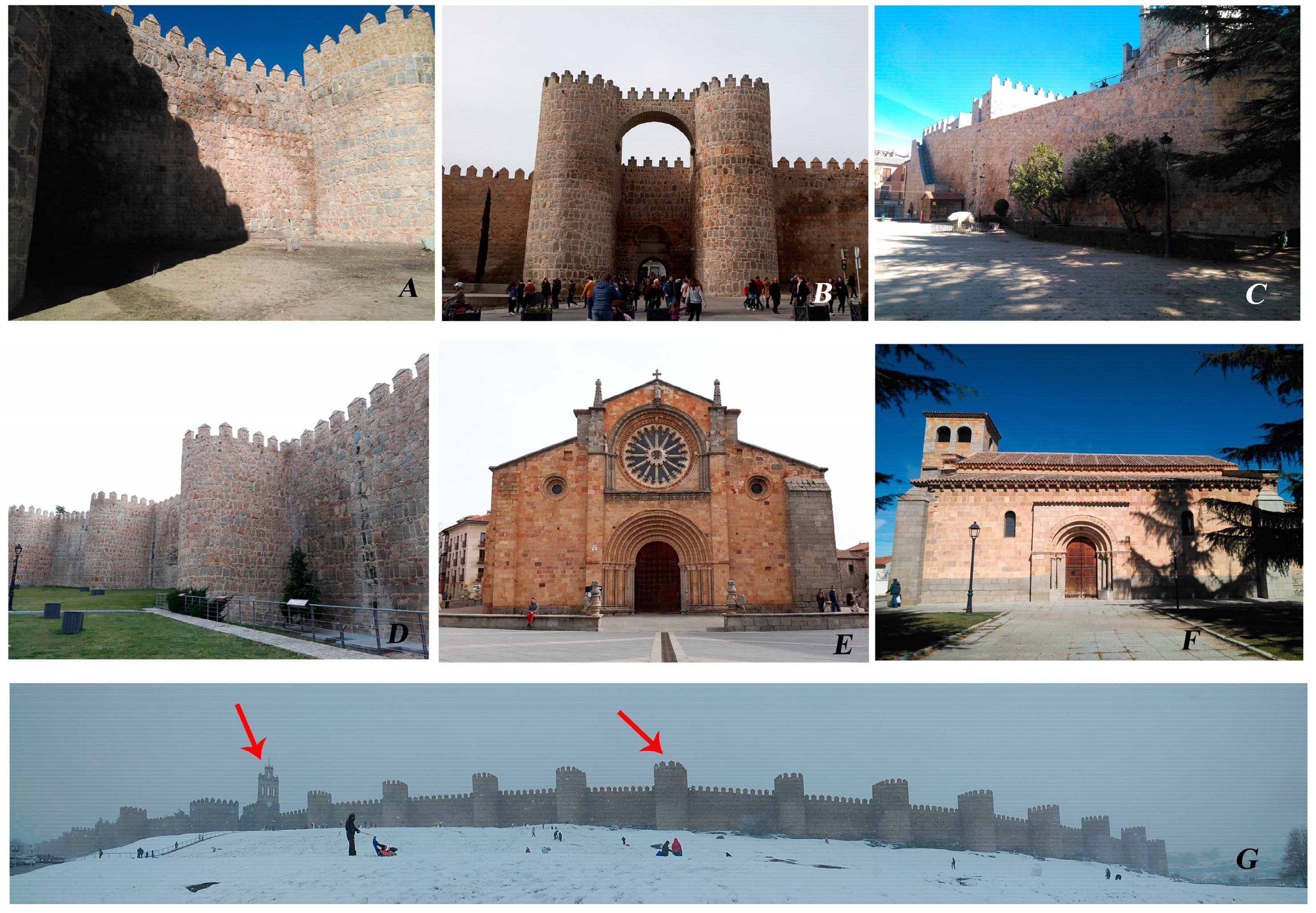The image depicts a collage of seven photographs, each labeled A through G. The arrangement consists of two rows of three photos each (A-F), and one wide, horizontal photo at the bottom (G). The majority of the photos (A to F) capture various views of a castle-like structure with impressive stone walls and crenellations. Photo A shows an interior section of the castle, while B features two prominent columns from the exterior. Photos C and D offer side views that emphasize the large scale of the structure. However, photos E and F shift focus to buildings that resemble a church and its rectory, suggesting different architectural styles within the same vicinity. The bottom photo, G, portrays a long, snow-covered wall with fortress-like towers, possibly indicating the Great Wall of China or a similar historic fortification. Two red arrows point to specific parts of the wall, and children can be seen sledding down a snowy hill in the foreground. The collage weaves together various perspectives and styles of what appears to be a historical castle complex.